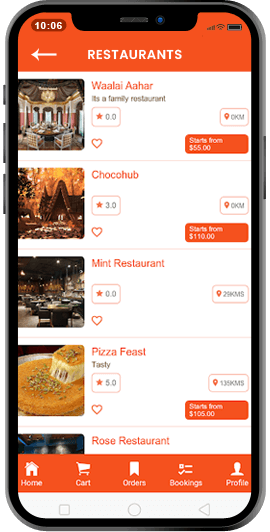The photograph displays a smartphone with an app interface superimposed onto its screen. The phone is set against a plain white background, featuring a metallic edge. The device is oriented in portrait mode and has rounded edges. A close examination reveals that this phone image is likely a graphical representation rather than an actual physical phone.

At the top of the screen, there is an orange header segmented by a horizontal line. Within this header, a reddish text bubble contains the number '1006,' accompanied by icons indicating network signal strength, Wi-Fi signal, and battery life. Below, on a white background, the word 'Restaurants' is displayed along with a back arrow situated on the left.

The app appears to be a restaurant listing service, with each entry featuring an image, name, star rating, favorite icon (heart), and starting price. The first listing showcases an outdoor seating area with a table. It is named "Walei Ahar" and labeled as a family restaurant. This entry has zero stars, implying it is unrated, and a heart icon next to it. The starting price is indicated as $55.

Subsequent listings include:
- "Choco Hub": This establishment has a three-star rating and a starting price of $110.
- "Mint": This entry lacks a star rating and starting price information.
- "Pizza Feast": Labeled as 'tasty,' it boasts a five-star rating with a starting price from $105.
- "Rose Restaurant": This entry does not provide any rating or starting price details.

All the listings follow a consistent format, presenting a cohesive and user-friendly visual layout.